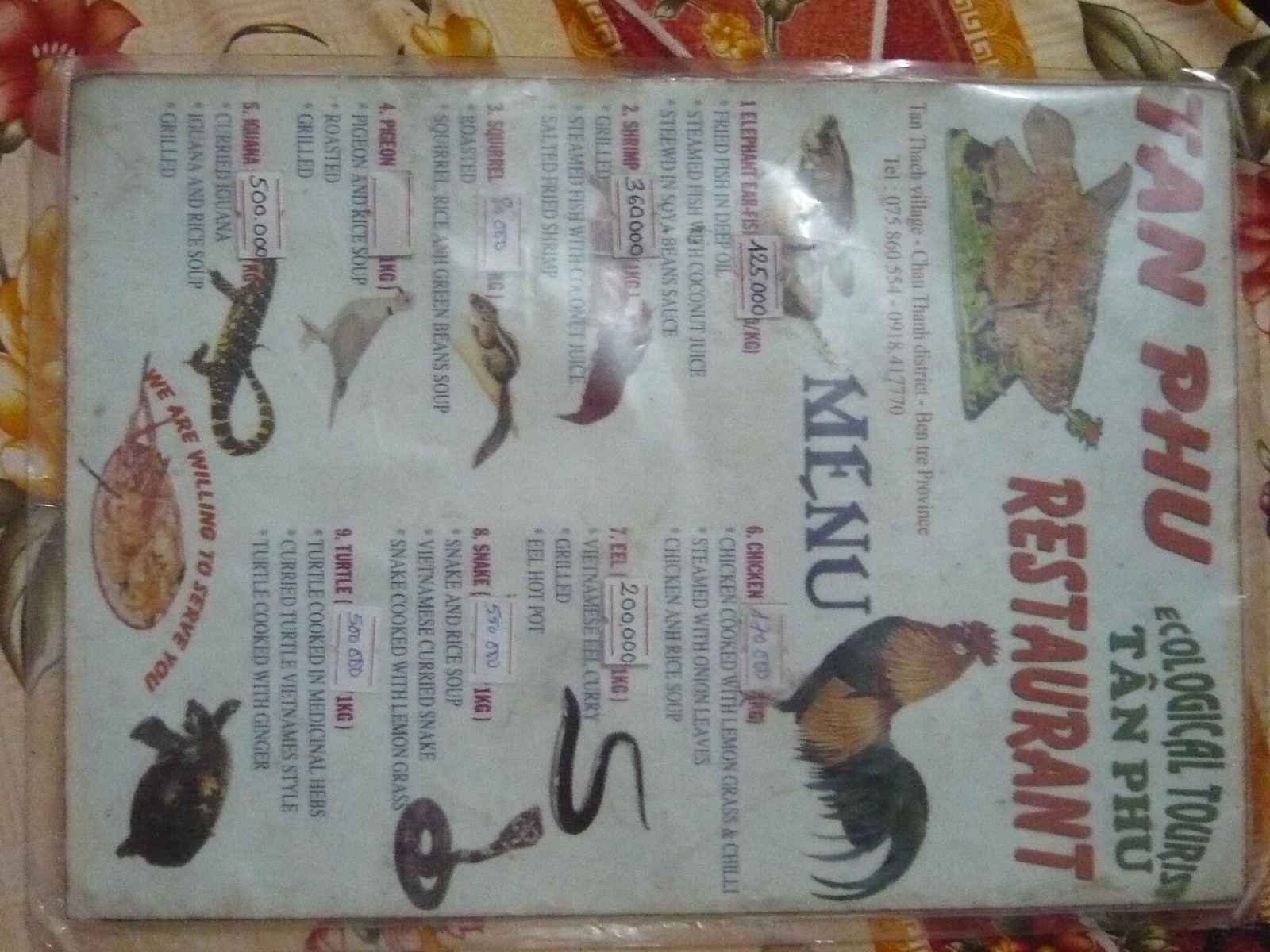The image depicts a horizontally oriented menu from Tan Fu Restaurant, titled "Ecological Tourism Tan Fu" in bold red text. The menu is tilted 90 degrees to the right, making the text appear vertical. On the right side of the cover, there is an illustration of a chicken, along with the word "Menu." The menu lists various exotic meats with their prices in a foreign currency. The animals featured include fish, a squirrel, a snake with a small sly cobra, a turtle at the bottom right, an iguana, and a pigeon. The menu is laid out on a table, emphasizing the restaurant's focus on serving a diverse range of animal species.